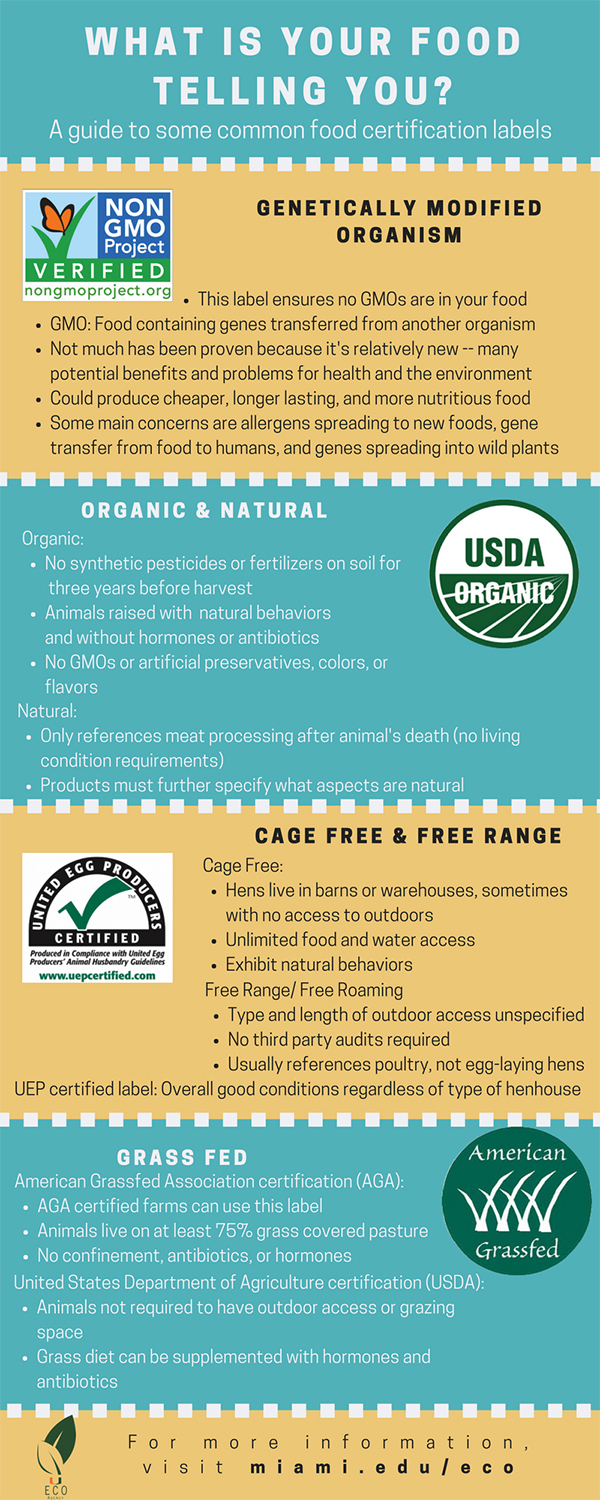The image is a vertically oriented, rectangular infographic, designed to serve as an informational card explaining various food certification labels. At the top, bold white letters announce the title, "What Is Your Food Telling You? A Guide to Some Common Food Certification Labels." The infographic is segmented into four main sections, each distinguished by alternating turquoise blue and light orange rectangles with corresponding text in contrasting colors—white print on turquoise and black print on light orange.

The first section is dedicated to "Genetically Modified Organism (GMO)" and features a "Non-GMO Verified" label. The second section explains "Organic and Natural" labels, highlighted by the USDA organic certification. The third section covers "Cage-Free and Free-Range" labels, while the final section focuses on "Grass-Fed" certifications.

Each section provides detailed descriptions of these labels, set apart by small white square dividers. At the very bottom, the infographic invites viewers to visit a website, specified as "miami.edu/eco" for more information. The overall design is both educational and visually structured to aid consumers in understanding food certification labels when making purchasing decisions.